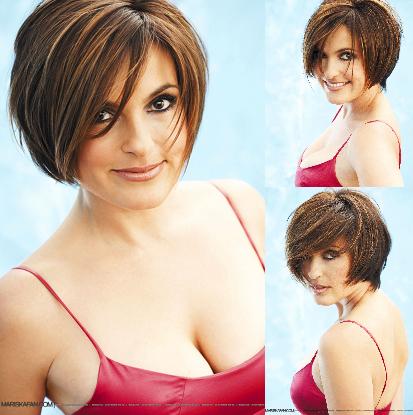The image features three distinct photographs of a woman with short, brown pixie-cut hair and smoky eye makeup, accentuated with black eyeliner and mascara. The background is a light sky blue. The composition of the image is divided such that approximately 65% of the left side displays a full-length view of the woman, who is wearing a red tank top with thin straps, showing a lot of skin and a bit of cleavage. She is smiling softly and staring directly at the viewer. 

On the right side, the remaining portion of the image is split horizontally into two equal parts. The top right section shows the woman again, smiling confidently with her teeth visible and gazing at the viewer. The bottom right section captures her with a neutral expression, still looking outward. The red tank top appears slightly leathery, and the woman's overall appearance exudes confidence and poise in all three photographs.